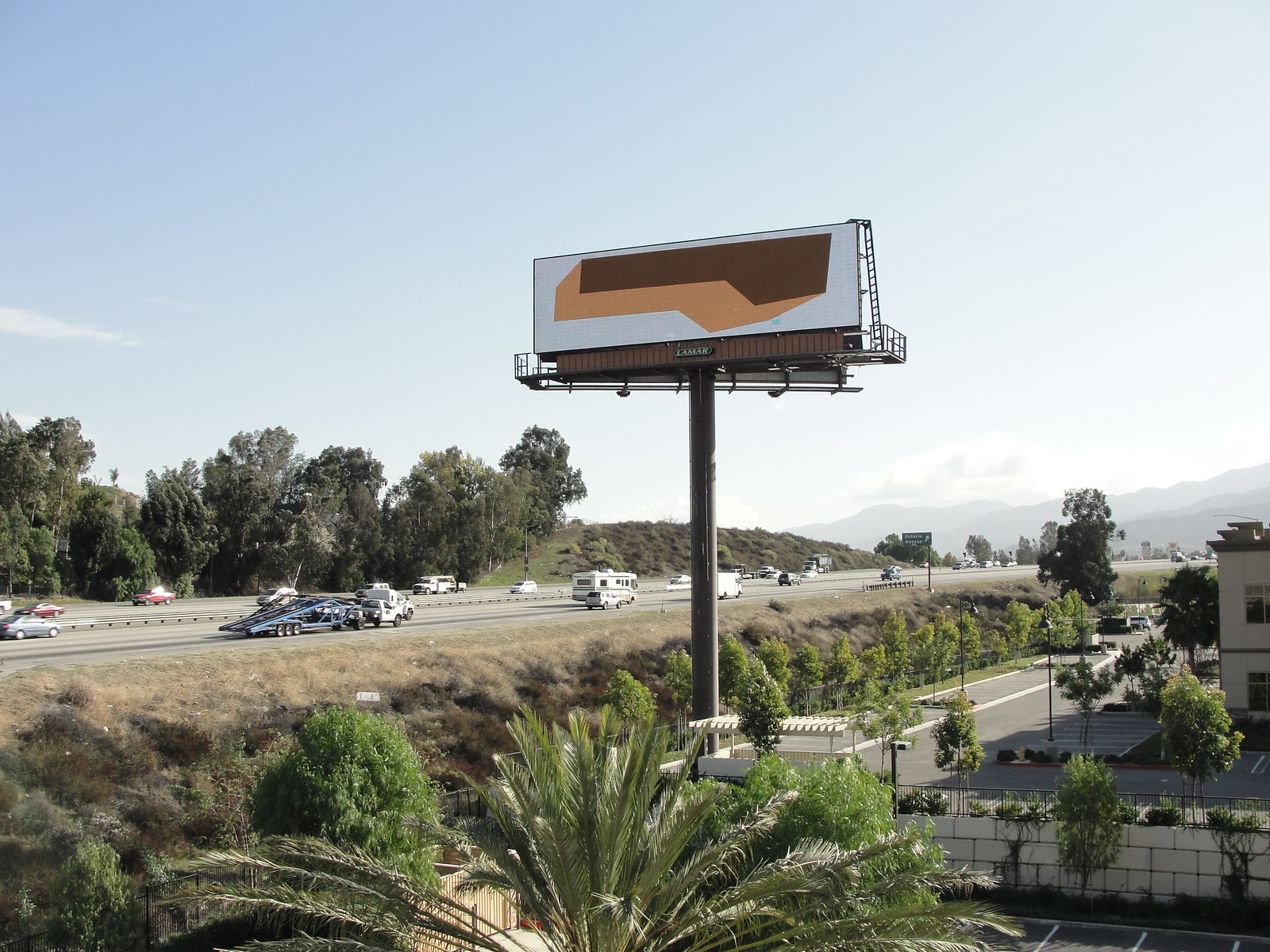This daytime photo captures an expansive outdoor scene taken from a property adjacent to a freeway, visible in the distance running horizontally from left to right. The foreground is characterized by a parking lot dotted with neatly arranged palm trees and landscaped bushes. Prominent in the middle ground is a building surrounded by more decorative greenery, adding a touch of sophistication to the area. Additionally, there's a large, empty billboard structure, likely pending new advertisements, standing tall with a rectangular sign extending upwards. In the far background, majestic mountains rise beneath a partly cloudy blue sky, completing the picturesque setting.